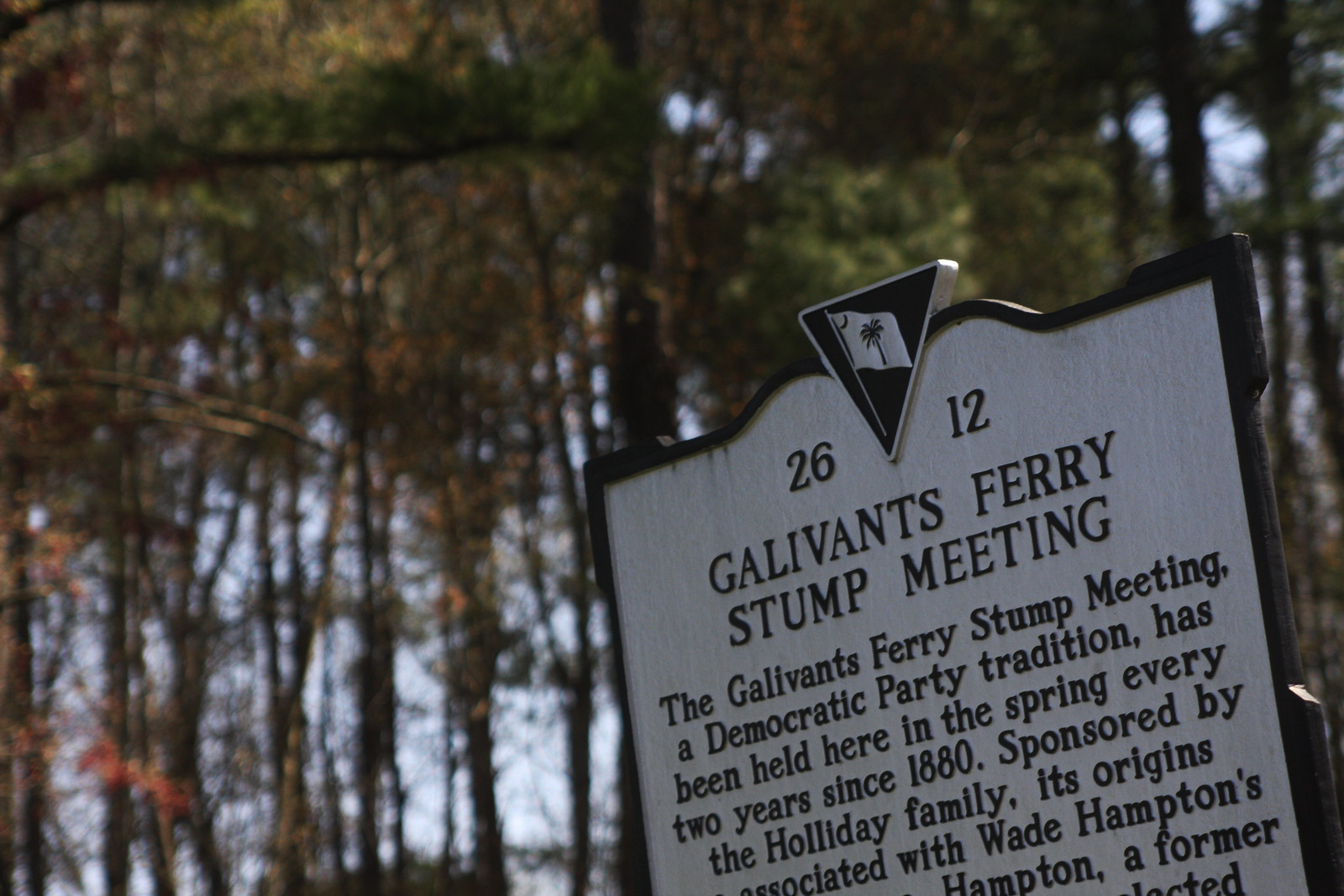In this outdoor daytime photograph, a historic memorial placard is prominently displayed in the bottom right corner at a tilted angle. The placard features a black-outlined metal sign with an upside-down triangle logo at the top, inside which is a white flag adorned with a palm tree. Flanking the triangle, the numbers "26" and "12" are visible. The sign bears the title "2612 Gallivant's Ferry Stump Meeting" and provides a brief historical note: "The Gallivant's Ferry Stump Meeting, a Democratic Party tradition, has been held here in the spring every two years since 1880, sponsored by the Holladay family, its origins associated with Wade Hampton." The text cuts off after "Hampton, a former," due to the angle of the photograph. The background is a natural, wooded area with tall trees and patches of blue sky visible through the foliage. The upper part of the image is filled with tree tops in various shades of green, gold, and red, while the lower section reveals tree trunks with light filtering through them, adding to the serene, historic ambiance of the setting.